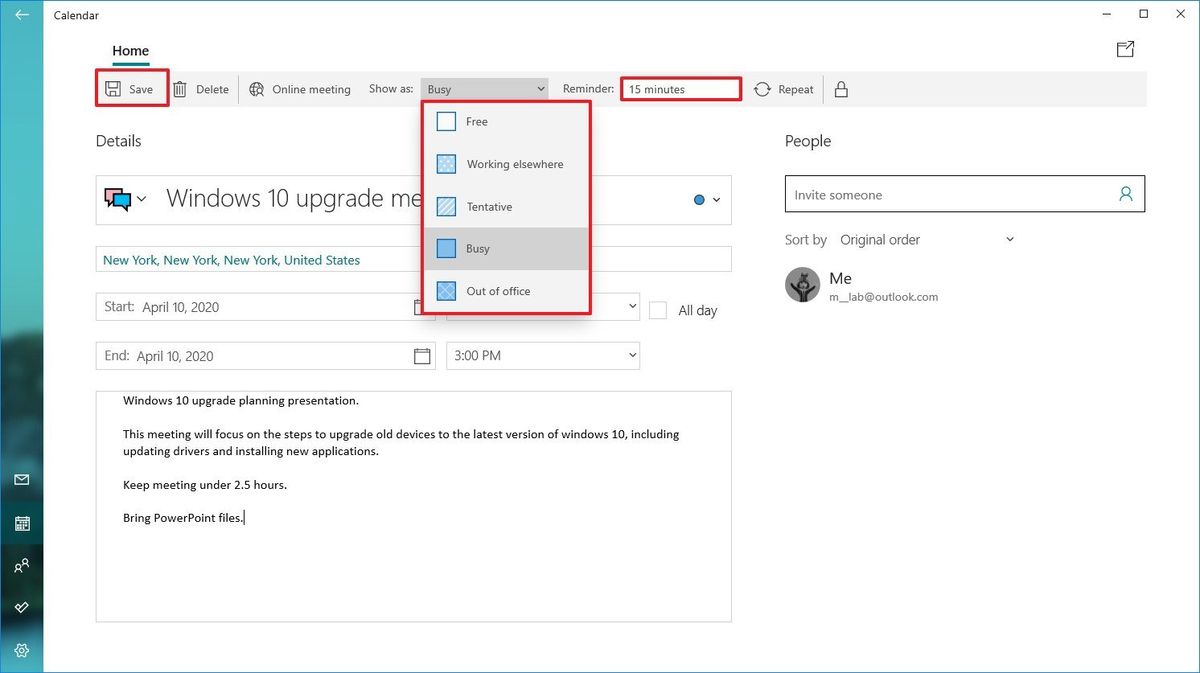On a white background, the image features a detailed digital scheduling interface. 

**Left Side:**
- A prominent vertical blue box with dark blue and black text. 
- A white left arrow at the top.
- Five white icons at the bottom.
- A calendar within a white section.

**Top Right:**
- Several small icons: a blank square, an X, and a small box with an upward-right arrow.

**Middle Section:**
- Options starting with "Home" underlined in blue.
- A red box around "Save," followed by "Delete."
- Labels for "Online meeting," "Show as," and "Busy."
- Drop-down menu with statuses: "Free," "Working Elsewhere," "Tentative," "Busy," and "Out of Office," each with a square outline.
- "Reminder" and a red box around "15 minutes."

**Bottom:**
- "Repost" followed by a lock icon and a blank field.
- "Details" section with a large split block: one side blue, the other pink, including a down arrow and text "Windows 10 upgrade," a blue circle, and another down arrow.
- A "People" section accompanied by a search menu.
- "Sort by original order" with a circle icon featuring a character and labeled "Me."
- Address details.

**Body Content:**
- "New York, New York, New York, United States."
- Event time: "Start April 10th, 2020" and "End April 10th, 2020."
- Calendar icon next to "3 o'clock PM," with an "All day" option above.
- A meeting description box: "Windows 10 Update Planning Presentation." Mentioning the focus on upgrading devices, updating drivers, and installing applications, with instructions to keep the meeting under 2.5 hours and bring PowerPoint files.
- A line at the bottom.

Overall, this image represents a comprehensive and meticulously detailed digital meeting schedule or planner.